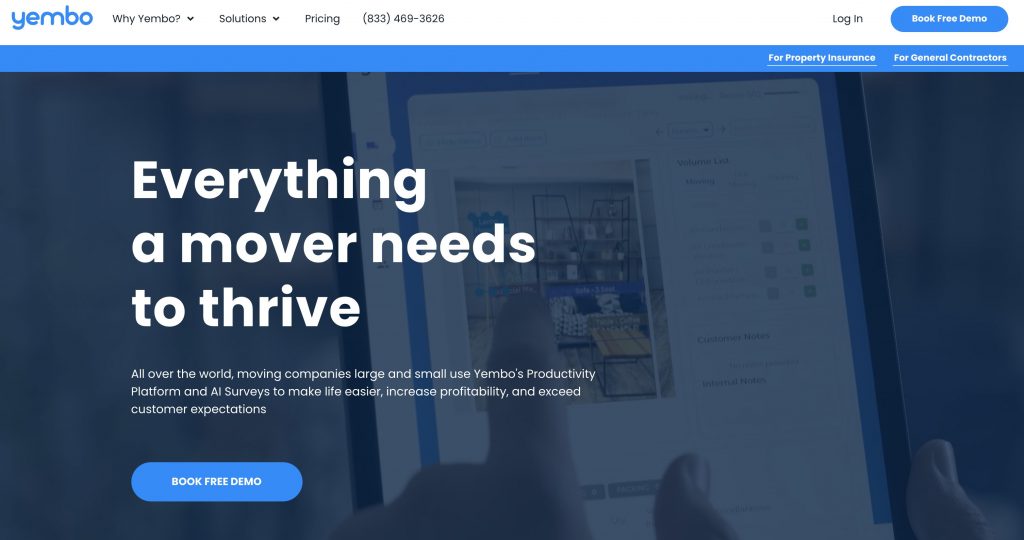This image is a homepage screenshot from a website called Yumbo. Across the top of the page, there's a white navigation bar with links labeled "Solutions" and "Pricing," and the company's phone number. Further to the right, there is an option to "Log In" and a prominent blue button that invites visitors to "Book Free Demo."

At the far right of the navigation bar, within a blue rectangle, there are clickable options for "For Property Insurance" and "For General Contractors." Below the navigation bar is a dark, semi-transparent navy rectangle. In the background of this section, a person is holding a tablet and pointing at something displayed on it.

In the foreground, white text declares, "Everything a Mover Needs to Thrive," followed by a detailed description: "All Over the World Moving Companies Large and Small Use Yumbo's Productivity Platform and AI Surveys to Make Life Easier, Increase Profitability, and Exceed Customer Expectations." Another blue "Book Free Demo" button is prominently displayed below this text.